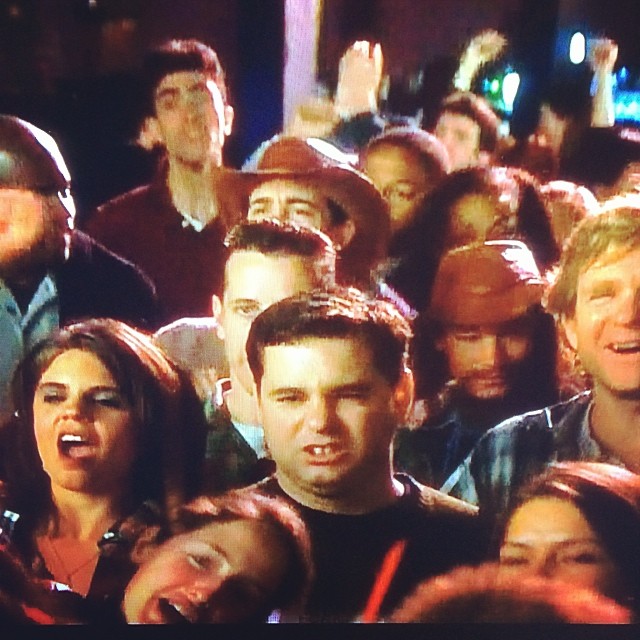In this evocative scene, we encounter a stylized crowd reminiscent of a movie set. The individuals, predominantly light-skinned, exude a range of intense emotions. Center-right, a blonde man in a plaid shirt of purple and light blue appears to be almost laughing. Beside him to the left is a man with a serious and downcast expression, distinguished by his red leather-like baseball cap and light mustache.

On the left side, a woman with dark hair is seen yelling vehemently, her mouth agape revealing the top teeth and tongue, her eyes predominantly closed. She wears an open blouse that reveals a thin gold necklace around her neck. To her right, another person with light blondish hair leans over, also yelling.

Among this animated crowd, several noteworthy figures stand out: near the center-left, one person dons a red cowboy hat while looking upward, and in the back center, partially obscured, is an individual with almost shaved hair.

The collective display of emotions, from anger to amusement, captures a vivid moment of human interaction and drama.